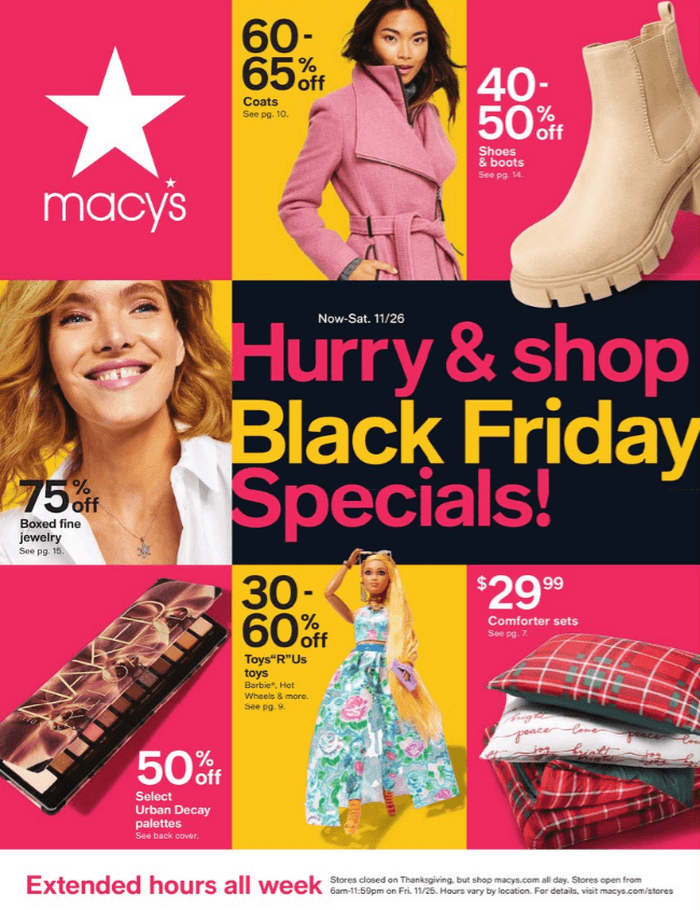This image is an advertisement from Macy's promoting their Black Friday specials. The design features four corners with a reddish-pink hue, framing the visual composition. At the top and bottom center of the image, there are two sections with a yellow background. Dominating the middle is the standout element: a photograph of a smiling woman. Surrounding the woman's image is a central black box highlighting the top Black Friday deals.

At the very top, a star is prominently displayed next to the Macy's logo. Adjacent to this, text against a yellow background announces "60 to 65% off coats." Next to it, the ad communicates "40 to 50% off shoes and boots." 

Centered within the black box, near the smiling woman, there's a highlight for "75% off boxed fine jewelry," with a note prompting viewers to "see page 15" for more details. 

The headline, "Hurry and shop Black Friday specials," urges immediate action. Towards the bottom segment, more exclusive deals are outlined: "50% off select Urban Decay palettes," "30 to 60% off Toys R Us toys," and a special price of "$29.99 for comforter sets." The diverse layout and vibrant colors emphasize the urgency and variety of the Black Friday offers at Macy's.